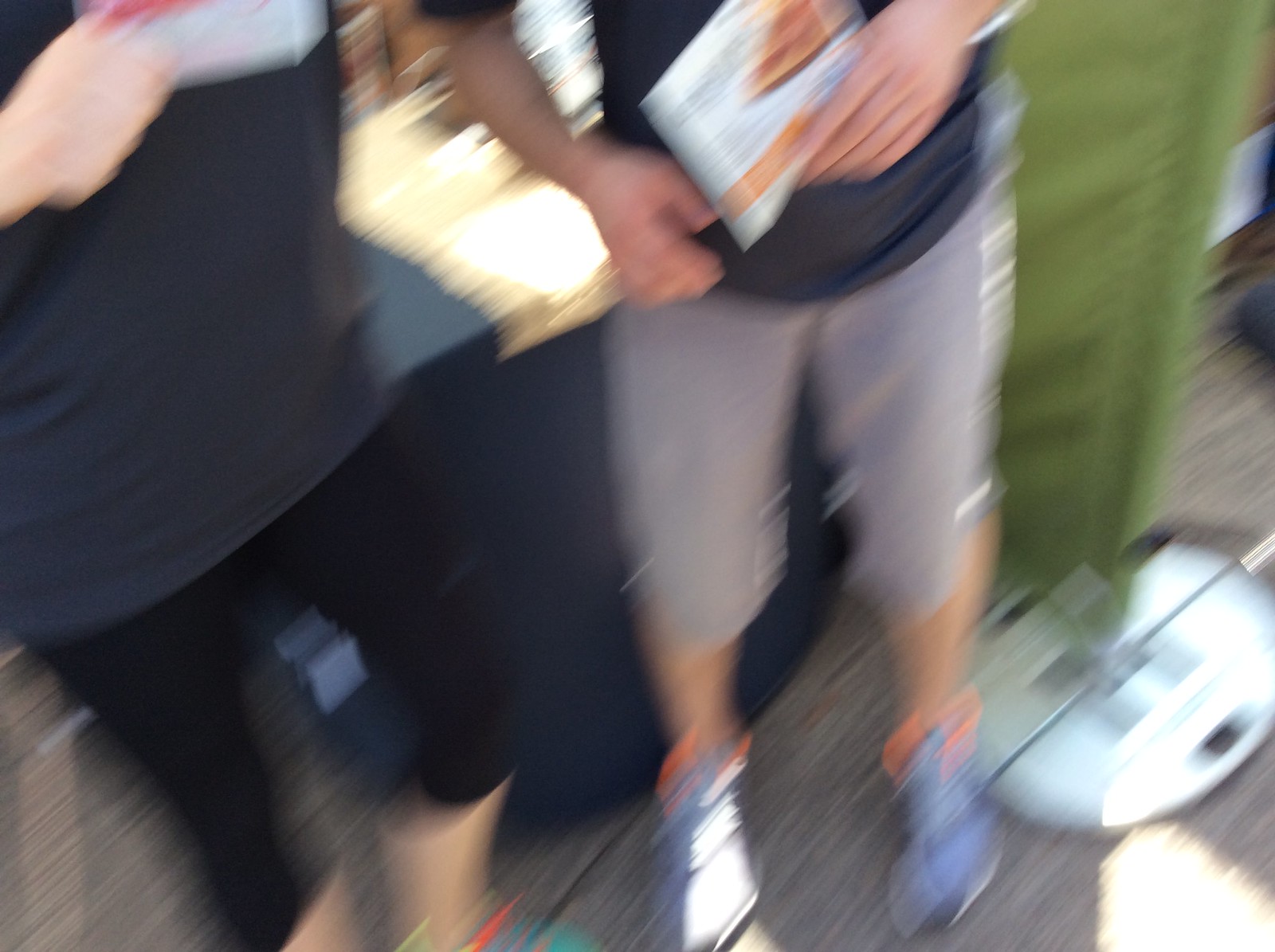In this blurry photograph, two Caucasian individuals are partially visible, with only their torsos and lower bodies in the frame. The person on the far left is dressed in a short-sleeved gray t-shirt and tight-fitting black pants. The individual standing next to them is similarly wearing a short-sleeved gray t-shirt paired with light-colored, knee-length shorts. Both appear to be in grayish tennis shoes with subtle orange details. The background features a greenish-colored curtain.